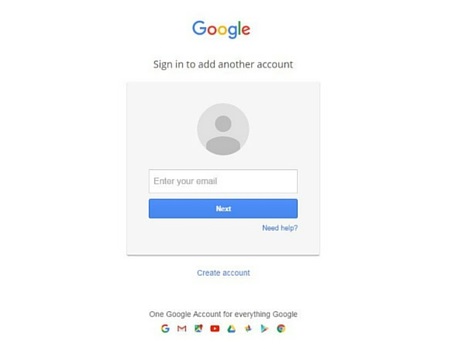This screen capture depicts a Google account sign-in page. Prominently displayed at the top is the multi-colored Google logo encompassing shades of blue, red, gold, and green. Below this, the prompt "Sign in to add another account" is rendered in gray text. Adjacent to this text, a gray circle featuring a small person icon is visible.

Centrally, a white sign-in box invites action with the instruction "Enter your email" in light gray text. Beneath this, a blue rectangular button containing the white word "Next" is shown, ready for interaction. On the left, in blue font, the phrase "Need help?" accompanied by a question mark offers assistance.

Emerging from the lower section of the gray area, the option to "Create account" appears in blue text. Further down, the statement "One Google account for everything Google" is printed in gray, highlighting the integration of Google's services.

At the bottom of the image, multiple icons representing various Google services are neatly arranged. From left to right, these include:
1. The multi-colored Google "G".
2. The red and white Gmail envelope.
3. The green, red, and blue Google Maps pin.
4. The red and white YouTube play button.
5. The green, yellow, and blue Google Drive triangle.
6. An indistinguishable icon due to its small size.
7. A pink and green triangular-form icon.
8. The iconic green, red, yellow, and blue Chrome circle, denoting the web browser. 

The screen capture is slightly blurry, causing some text to appear less legible, although the overall quality remains acceptable for interpreting the image content.